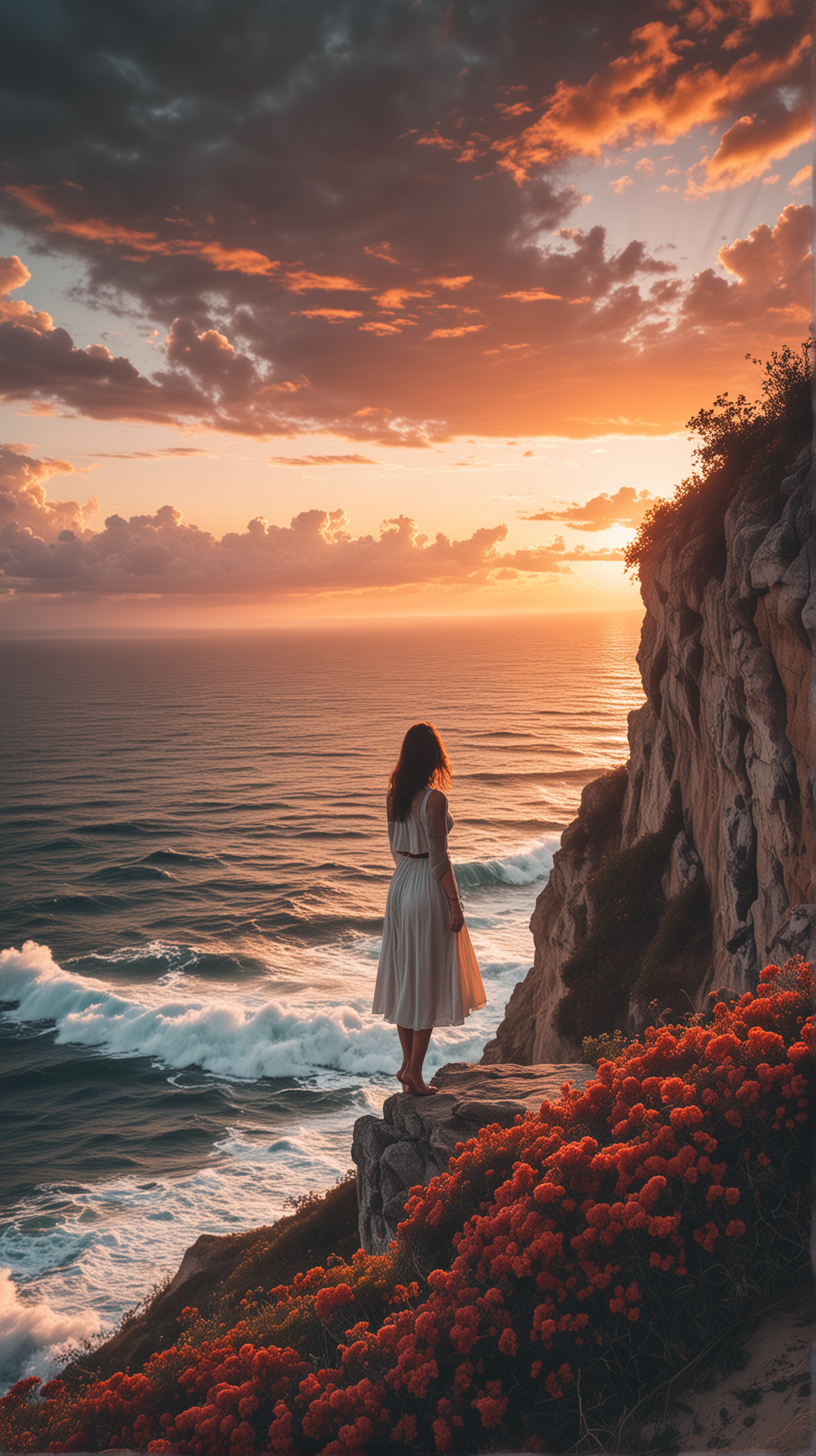The image features a high-quality, digitally created scene of a woman standing precariously on the edge of a rocky cliff, overlooking a vast, almost gray ocean. The woman, dressed in a beige dress, has shoulder-length brown hair and a light complexion. She stands barefoot, with her back mostly facing the camera and her body slightly angled. On her right arm, she wears a visible band, while her left arm is not visible. Surrounding her on the cliffside is a lush bed of vibrant red flowers, densely packed and almost cylindrical in shape. To her left, the waves crash against the cliff, their colors transitioning from dark to white and blue, creating a sea foam pattern that continues behind her. Above, the sky is mostly covered in gray clouds with sporadic gaps of cyan, tinged with accents of orange and red from either a sunrise or sunset. The light from the sun casts an orange and yellow glow on the ocean's surface, enhancing the picturesque scenery. To her right, a steep cliff adorned with silhouetted plants or flowers adds to the dramatic landscape.